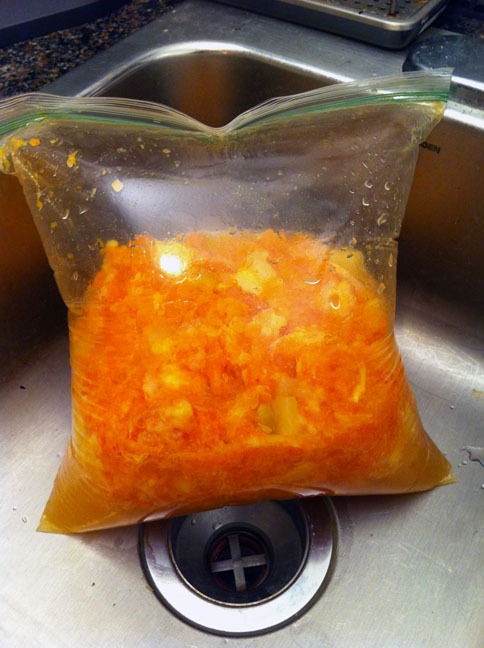In this detailed photograph, a medium-sized, transparent Ziploc bag with a green seal is placed inside a metallic, silver kitchen sink. The Ziploc bag, almost square in shape, appears poofy and swollen as if it's about to burst. It is partially filled, roughly halfway, with a semi-fluid, orange-red content that might be kimchi or something similar, creating visible gas buildup inside. The stainless steel sink is only partially visible, including the edge corner and the sink hole, but the focus stays on the bag seemingly ready to pop.